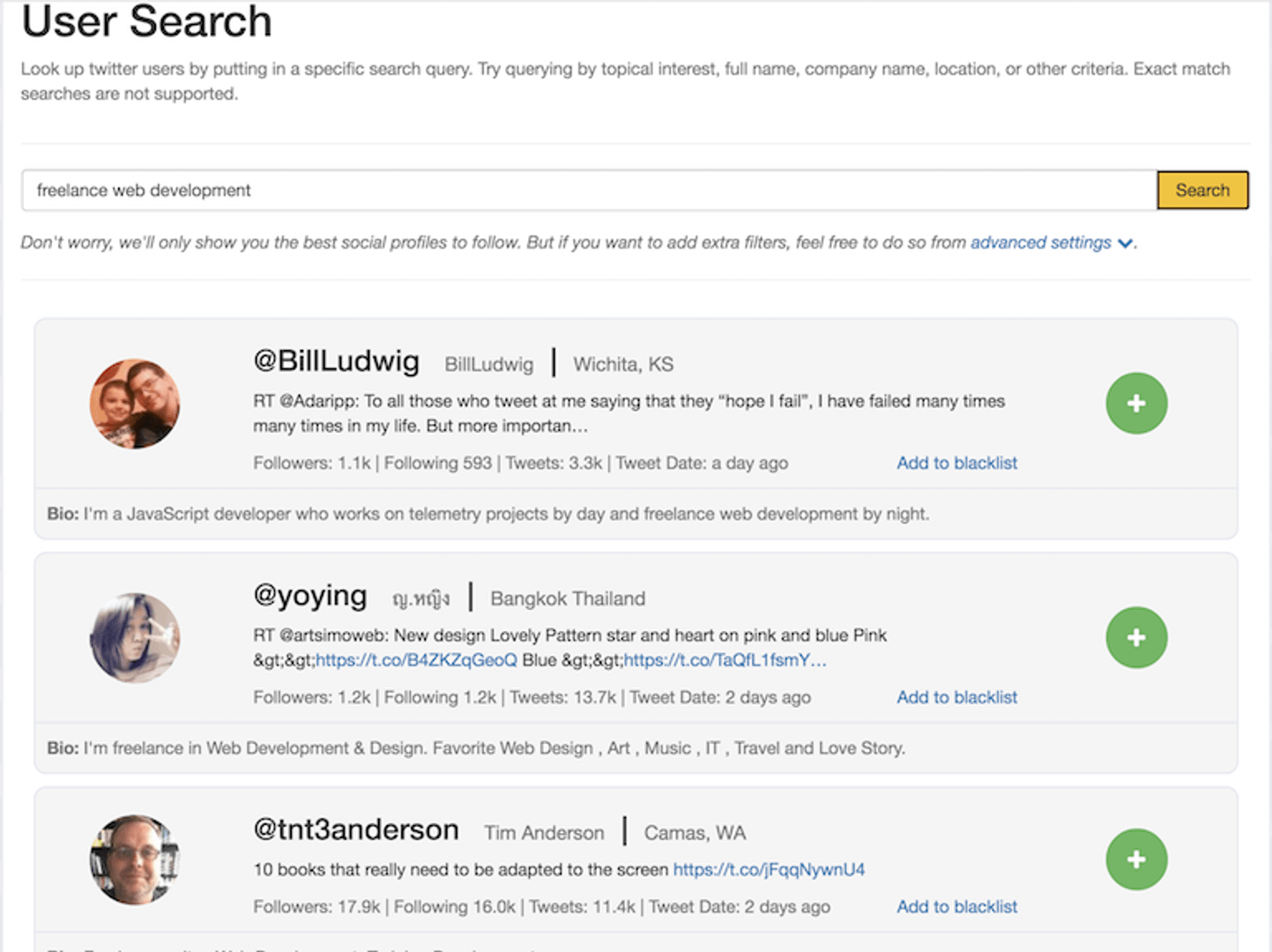Here's a cleaned-up and detailed caption based on the given voice input:

---

A Twitter search reveals a variety of users based on specific queries such as interests, names, companies, or locations. Key results include:

1. **Bill Ludwig from Wichita, Kansas**:
   - Followers: 593
   - Following: 1
   - Number of Tweets: 3.3k
   - Latest tweet: One day ago
   - Notable feature: Option to add to blacklist (indicated by a green circle with a plus sign)

2. **YeoYing from Bangkok, Thailand**:
   - Followers: 1.2k
   - Following: 1.2k
   - Number of Tweets: 13.7k
   - Latest tweet: Two days ago
   - Notable feature: Option to add to blacklist (indicated by a green circle with a plus sign)

3. **Tainterson, also known as Taint Anderson, from Camas, Washington**:
   - Followers: 17
   - Following: 18k
   - Number of Tweets: 11k
   - Latest tweet: Two days ago
   - Notable feature: Shared a list titled "10 books that really need to be adapted to the screen"
   - Option to add to blacklist (indicated by a green circle with a plus sign)

---